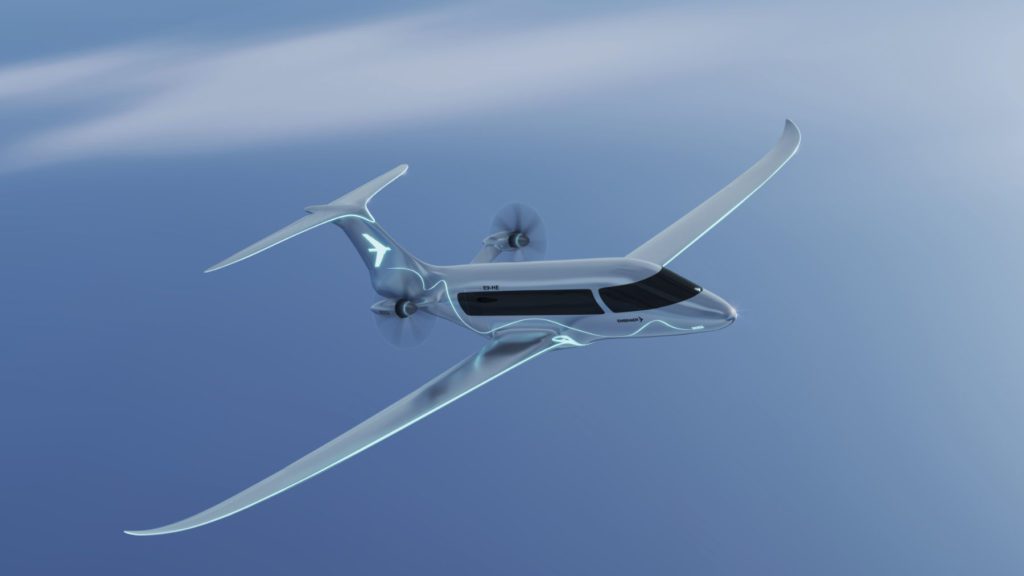This image, likely a computer-generated rendering, depicts a futuristic, sleek aircraft in mid-flight against a backdrop of a blue sky with wisps of light clouds. The metallic-looking jet features a continuous dark-tinted window that spans from the cockpit to nearly the tail, merging seamlessly to form a smooth, uninterrupted surface. It has two propeller-driven engines positioned near the tail, both slightly blurred to imply motion. The thin, sleek wings are devoid of any features underneath, terminating in tips that curve upward. The T-shaped tail displays a white silhouette of another jet, creating a striking visual echo of the main aircraft. The plane is banking gently, emphasizing its streamlined design and sophisticated appeal.